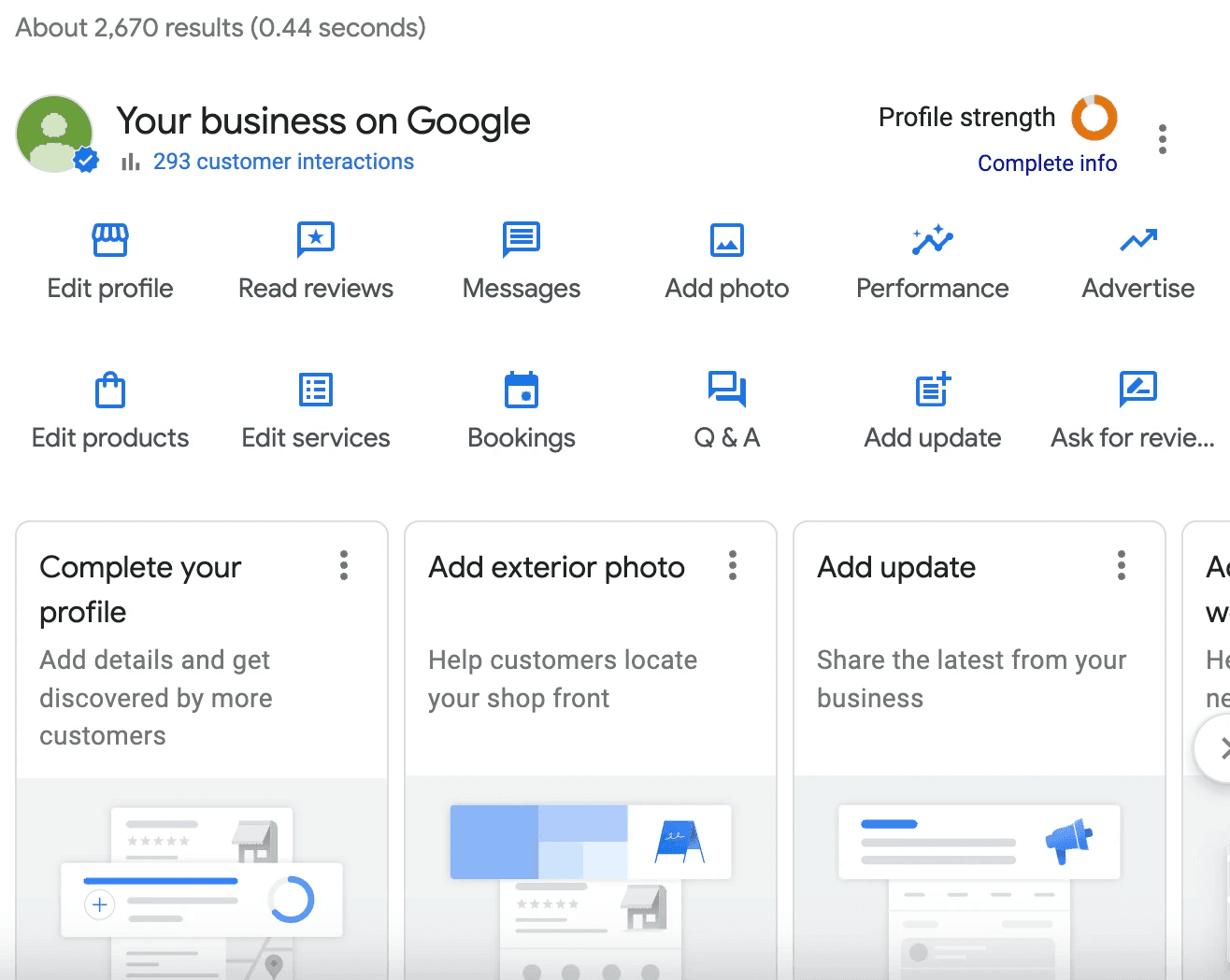This image is a detailed screenshot from Google My Business. In the upper left-hand corner, it shows a search result count of approximately 2,670 results. Just below this, there's a prominent section titled "Your Business on Google," highlighting 293 customer interactions. On the upper right-hand side, a "Profile Strength" indicator is displayed with an almost full orange circle, suggesting a near-complete profile.

Beneath these sections, there is a series of button options aligned on the left side of the screen. These options include "Edit Profile," "Read Reviews," "Messages," "Add Photo," "Performance," "Advertise," "Edit Products," "Edit Services," "Bookings," "Q&A," "Add Update," and "Ask for Review."

Below the main button options, there's a set of actionable prompts encouraging further profile completion. The first prompt says "Complete Your Profile: Add details and get discovered by more customers." The second prompt urges to "Add Exterior Photo: Help customers locate your shop front." The third section, slightly cut off, appears to encourage sharing updates from the business. There’s also a partially visible button aimed towards the right side of the screen.

Near the section labeled "Your Business on Google," a green profile icon is prominent, adding a visual cue to the screenshot.